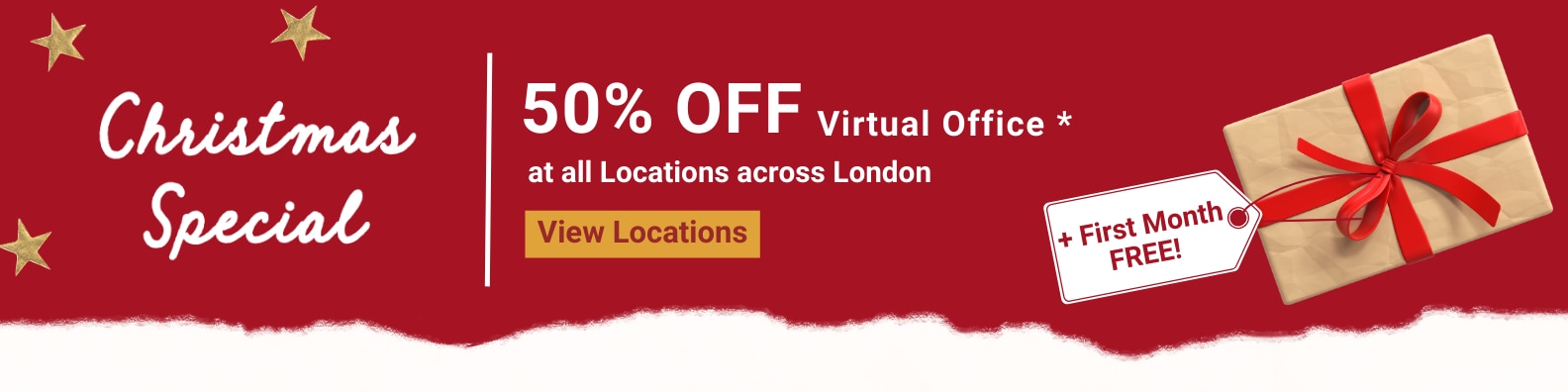The image is a partial screen capture of an advertisement from a webpage, promoting a Christmas special. The background features a maroon or reddish hue, providing a festive and warm atmosphere. On the left side, the words "Christmas Special" are elegantly scripted in white with "Christmas" positioned above "Special." Enhancing the seasonal theme, three gold stars are arrayed around the word "Christmas."

Dividing the text sections is a thin, vertical white line placed centrally. To its right, the advertisement boasts "50% off virtual offer*" in bold white text, followed by "at all locations across London" in a slightly smaller font. Beneath this information is a prominent orange rectangular button with red lettering, labeled "View Locations."

To the far right of the image, a bird's-eye view showcases a Christmas gift wrapped in luxurious gold paper, adorned with a striking red bow at its center. A white tag with red outlining attached to the gift proclaims "First Month Free."

The bottom edge of the image transitions with a shaded or faded white effect, giving it a soft, ethereal finish. Overall, the advertisement highlights a compelling holiday offer combining a 50% discount and a free first month, enticing viewers to explore the available locations.